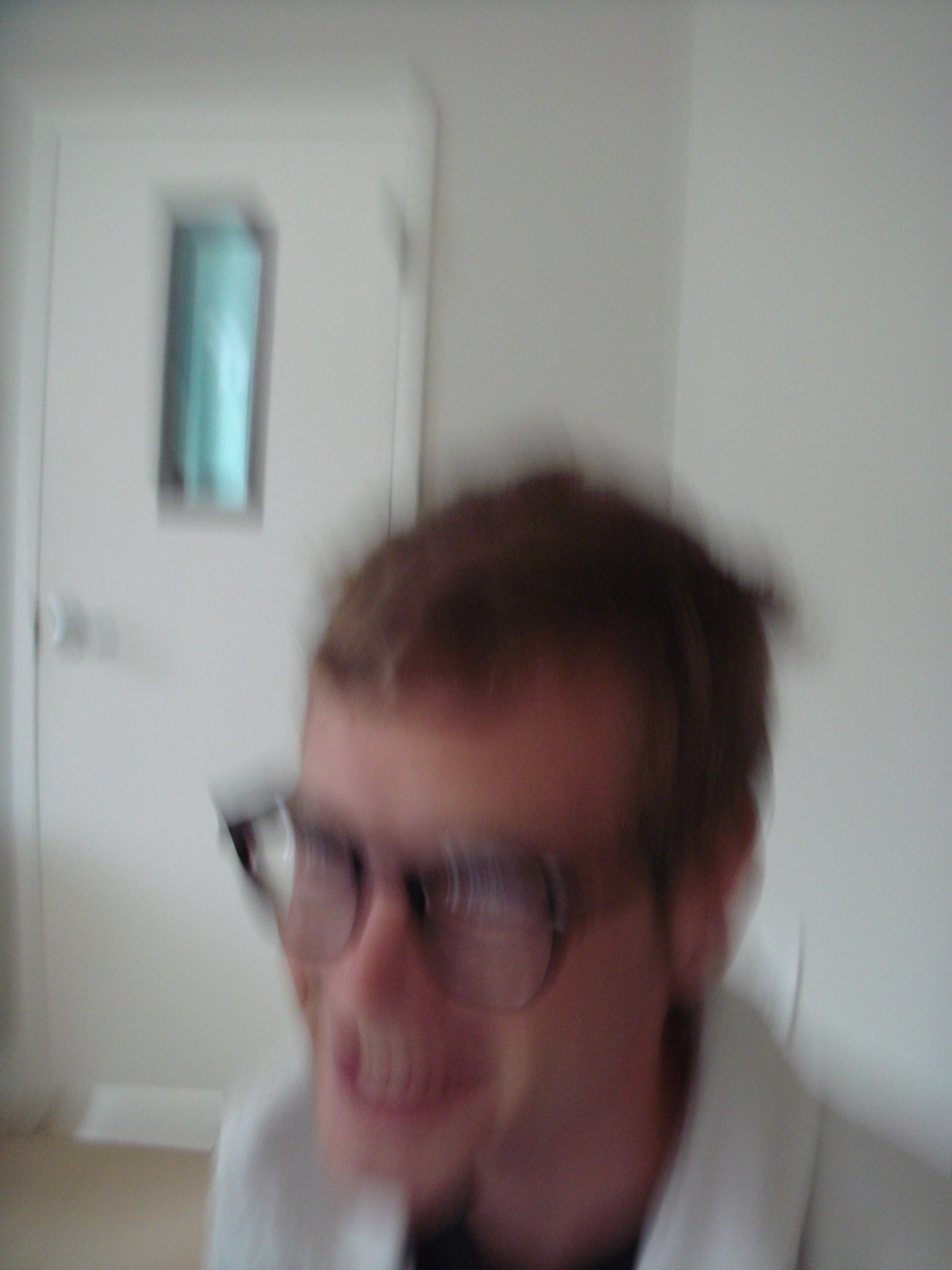This out-of-focus and blurry close-up photograph captures a white man with short unkempt sandy brown hair and pale skin standing in front of a white wall. He is adorned with dark, black-rimmed glasses and sports a very short, stubbly beard. The man is smiling, but the blurriness distorts his expression, making his large teeth appear almost exaggerated. He is dressed in a white jacket over a black shirt. In the background, to the left, there is a white door featuring a small, vertical, rectangular window at the top center, which casts a cloudy blue/turquoise hue. The presence of hinges and a handle suggest the door is meant for regular use, likely indicating that the setting is professional, possibly a scientific or medical workspace.